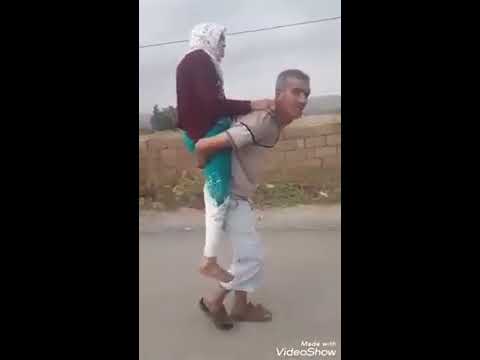This detailed photograph captures a man with brown skin, wearing a gray t-shirt, white capri-length pants, and brown sandals, carrying an older woman on his back. His arms are wrapped beneath her buttocks, supporting her legs. The woman, barefoot, is dressed in white pants and a greenish teal wrap around her waist. She sports a long-sleeved red cardigan sweater and a white scarf tied around her head. Her hands rest on the man's neck. This scene unfolds on a pavement or sidewalk, with a tan brick wall featuring shrubs and leaves at its base stretching behind them. Overhead, a power line hints at a cloudy day, adding depth to this image, which appears to be a still from a video.